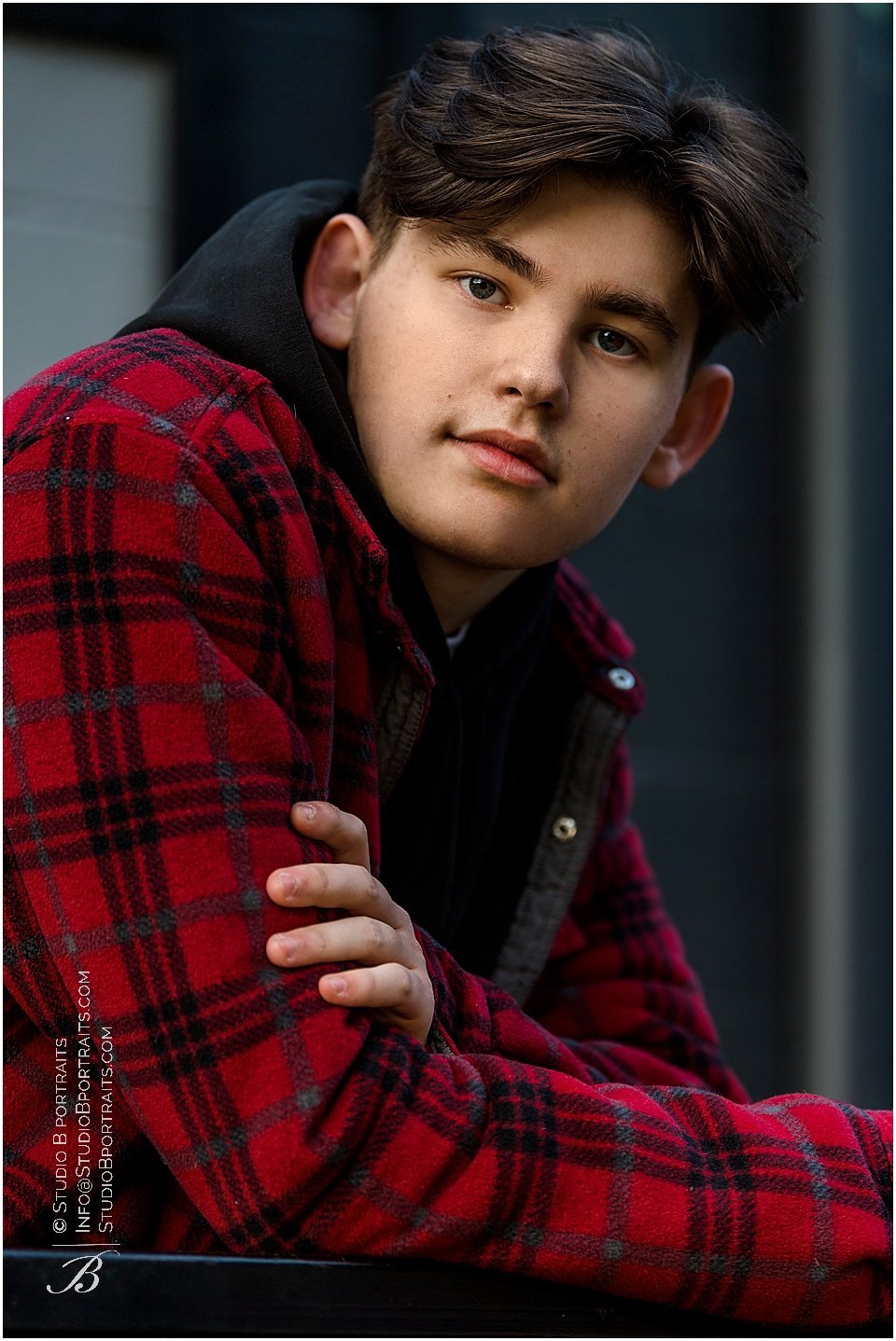This photograph features a young man, possibly a model, who is the primary focus of the image. He is wearing a vibrant red jacket adorned with black line designs, stripes, buttons, and it appears to be a hoodie. The young man is clean-shaven with stylish short black hair and thick eyebrows. He is slightly bent forward, with his hands resting on a metallic black railing. His intense gaze is directed straight into the camera, engaging viewers directly. The background of the image is blurred but hints at black and silver elements, possibly a wall or door. In the bottom left corner of the photograph, there is vertically oriented text reading "Studio B Portraits, info at studiobportraits.com, studiobportraits.com," accompanied by a B logo.